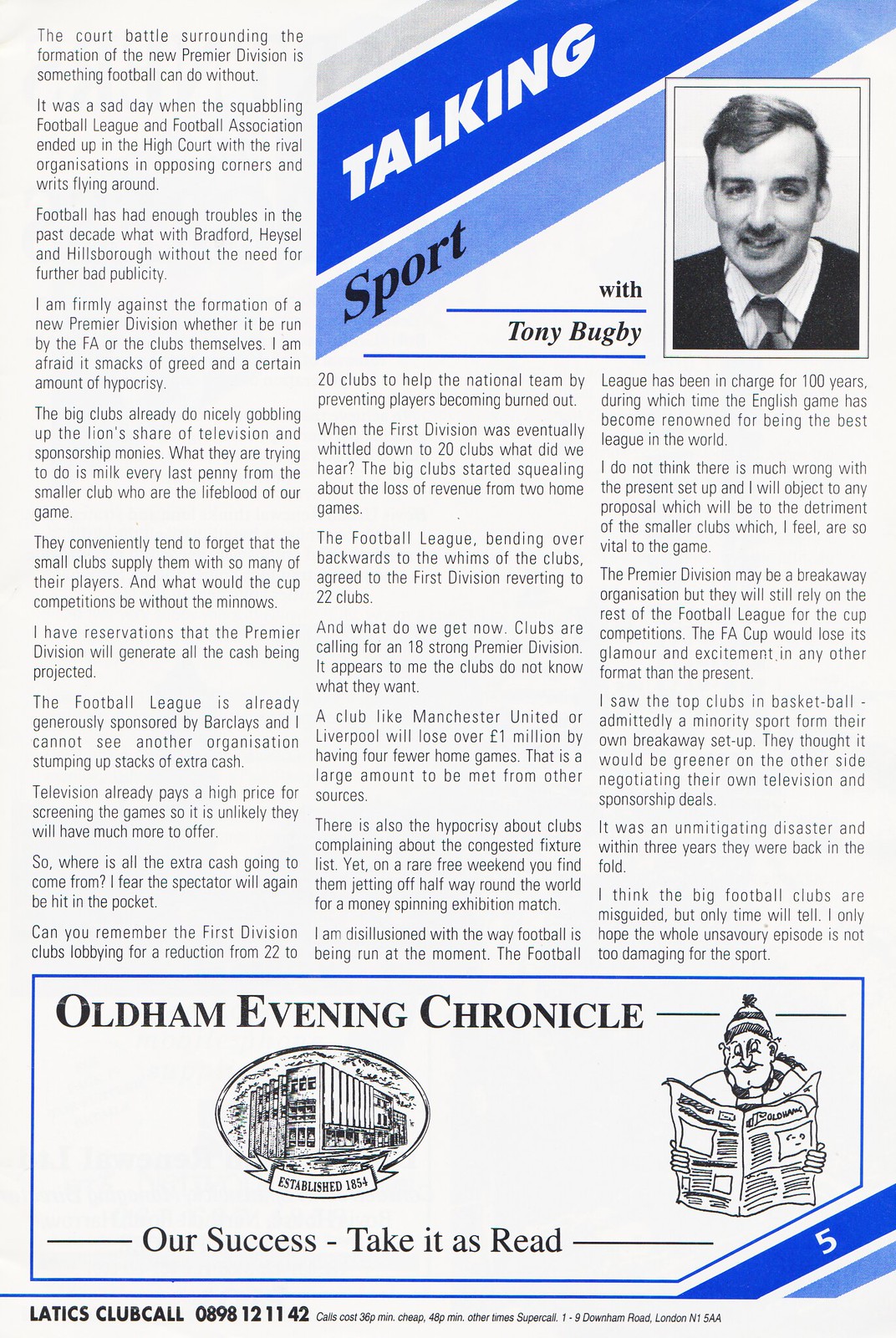This image depicts a page seemingly taken from a magazine or a newspaper. The background is white, and in the upper right-hand corner, there are two diagonal bars, one dark blue and one light blue. On the dark blue bar, the word "Talking" is written in white letters, and on the light blue bar below, the word "Sport" is in black letters. Adjacent to these, it says "With Tony Bugbee" in black text, followed by a thin horizontal blue line. To the right, there is a black and white photograph of a man named Tony Bugbee, identifiable by the caption. Tony is depicted wearing a dark sweater over a white shirt and tie, sporting short hair and a mustache, and smiling.

The main content of the page features a multi-paragraph article discussing sports, presented in three columns of text. The first paragraph begins with, "The court battle surrounding the formation of the new Premier Division is something football can do without."

At the bottom of the page, there is a blue box with the words "Oldham Evening Chronicle," accompanied by the slogan, "Our Success, take it as read." Adjacent to this text is a cartoon image of a man in a wool cap, reading a newspaper. Additionally, there is an oval logo with a sketch of a building and the text "Established in 1854" visible. In the lower right corner, another blue diagonal banner displays the number "Five," which likely indicates the page number rather than the cost.